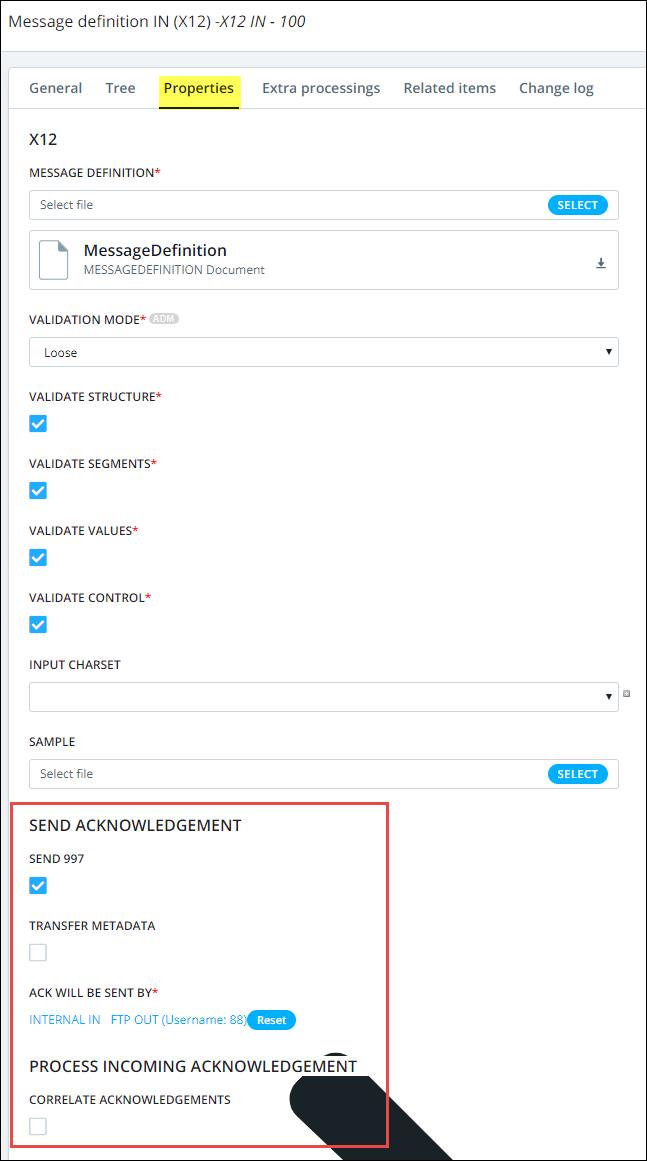The image depicts a detailed interface of a message configuration page titled "Message Definition [IN X1, 2, (numbers)]". The interface has multiple section headings including "General," "Tree," "Properties," "Extra Processing," "Related Items," and "Change Log," with the "Properties" section currently highlighted in yellow.

Beneath this, another heading reads "Message Definition," followed by a subsection labeled "Validation Mode," which is set to "Loose." The subsections "Validation Structure," "Validation Segments," "Validation Values," and "Validation Control" are all marked with a white check on a blue background, indicating they are selected.

The "Input Chart Set" field is empty, indicating no input has been provided. Additionally, there is a red box at the bottom labeled "Send Acknowledgement," and the "Send 997" option in a small blue box is checked. The "Transfer Metadata" option remains unchecked. A note indicates that an acknowledgment (ACK) will be sent by "Internal in PTP." The interface details are noted to be very small and difficult to read.